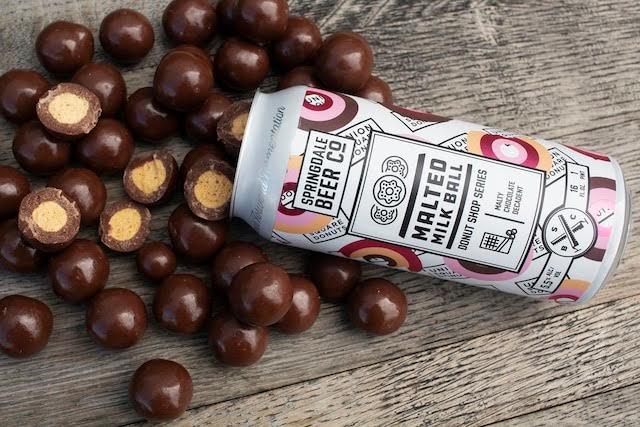This detailed photograph features an aluminum can of Springdale Beer, prominently labeled as part of their "Malted Milk Ball Donut Shop Series," with additional descriptors such as "Malted Milk Chocolate" and "Decadent." The beer can is decorated with an array of complex designs, including circular patterns that resemble bullseyes in red, pink, brown, and white, as well as numerous rectangular segments filled with text. Black symbols including starfish-like shapes and a railroad crossing with "SBC" for Springdale Beer Company are also visible.

The can is positioned on its side atop approximately 30 glossy, chocolate brown malted milk balls. Several of these milk balls are cut in half, revealing a tan, coffee-flavored nougat center. The entire arrangement rests on a vintage gray wooden table, which adds a rustic touch to the composition. Light reflects off the shiny surfaces of the malted milk balls, accentuating their texture and adding depth to the scene.